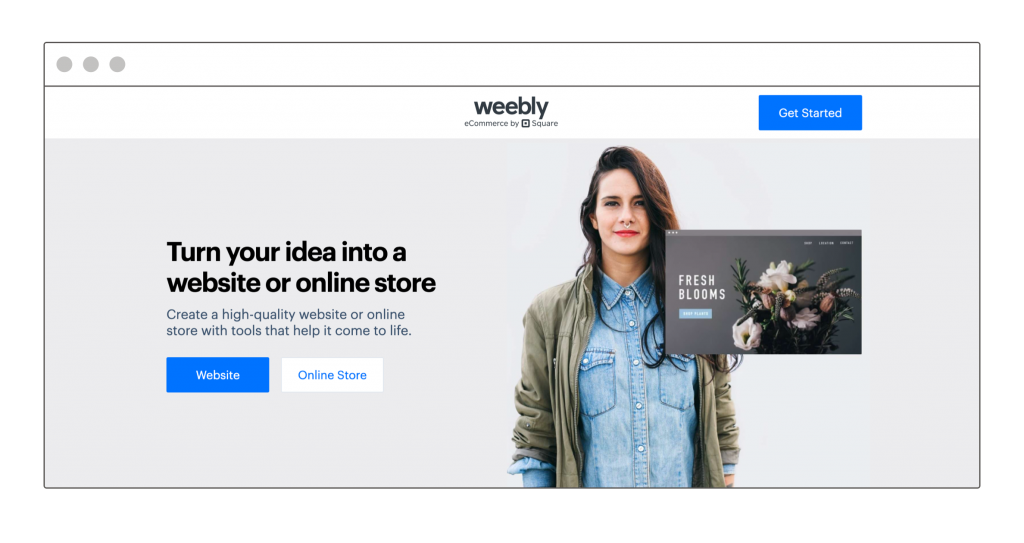This is a web page for Weebly, a website offering e-commerce solutions by Square. At the top center of the page, the logo "Weebly" is prominently displayed. To the right of this logo is a blue button labeled "Get Started." The background of the web page is a light gray color.

In the center of the page, there is an image of a woman with long brown hair. She has a silver nose ring and wears red lipstick. Her outfit consists of a blue denim button-up shirt and a light green khaki jacket. 

Overlaying this image in the upper right corner is an advertisement. The ad features a dark gray background with a bouquet of flowers in the center, and the text "Fresh Blooms" is prominently displayed. There is additional text below, but it is partially obscured and difficult to read, potentially saying "Start Plants Maybe."

On the left side of the page, black text reads: "Turn Your Idea into a Website or Online Store. Create a high-quality website or online store with tools that help you come to life." Below this text, there are two buttons; a blue button labeled "Website" and a white button labeled "Online Store."